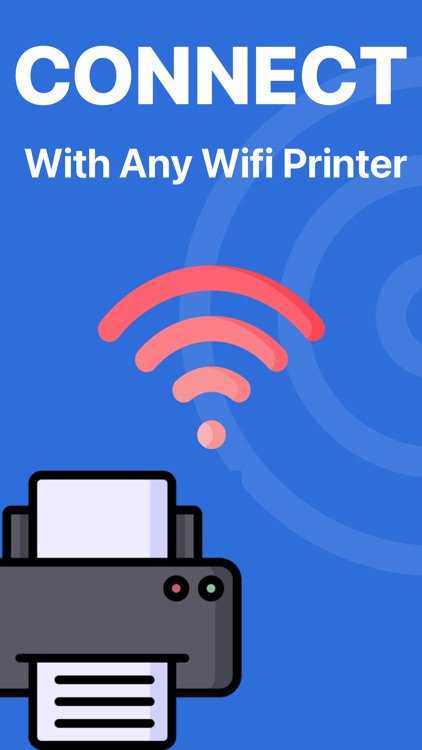The image is a detailed and vibrant diagram of a Wi-Fi printer, with the word "CONNECT" prominently displayed at the top in large white capital letters. Just below this in smaller capital letters is the phrase "With Any Wi-Fi Printer." Central to the diagram, beneath the text, is a red-colored Wi-Fi symbol consisting of three arcs and a dot at the bottom. Positioned towards the bottom left of the image is a realistic illustration of a gray printer, featuring both red and green LEDs. Paper is shown feeding into the printer and another paper sheet is depicted emerging with print on it. The entire diagram is set against a blue background adorned with subtle concentric circles positioned towards the right side.